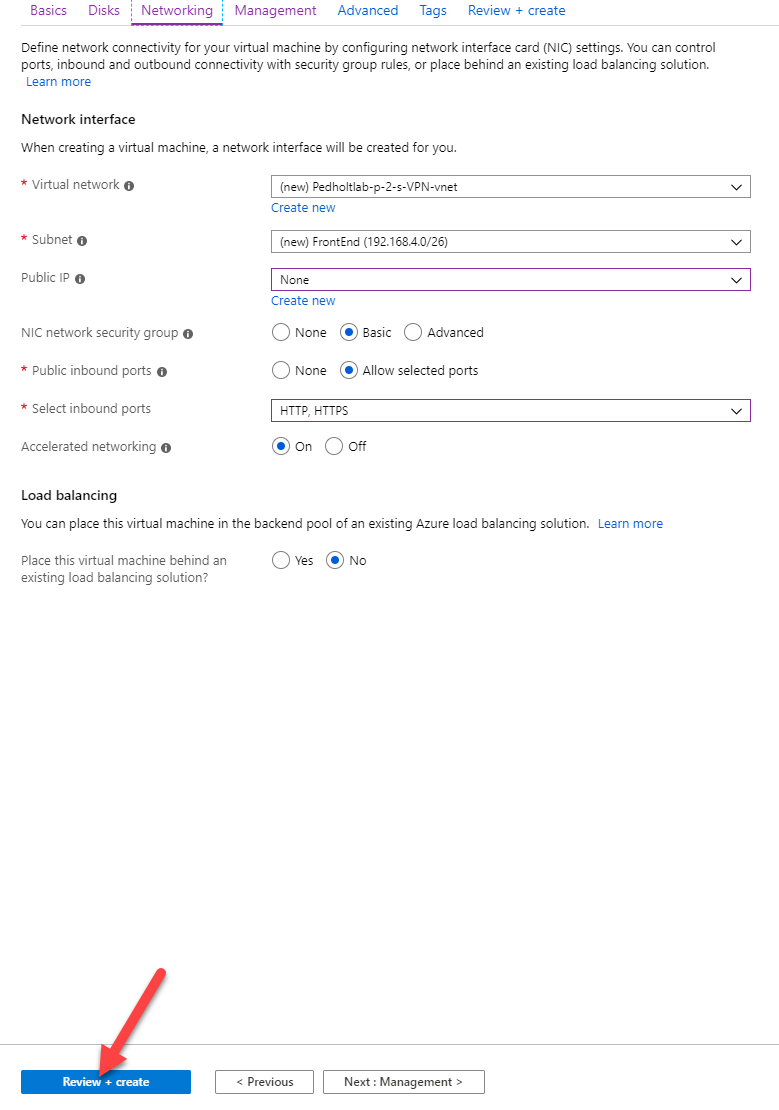This image is a screenshot of a web interface used for configuring a virtual machine's network settings. Set against a plain white background with no border, the interface features a navigation bar at the top with eight tabs: "Basics," "Disks," "Networking," "Management," "Advanced," "Tags," and "Review + Create." The first four tabs are in purple typeset, while the remaining three are in blue, indicating their clickable nature. The "Networking" tab is currently selected.

Beneath the tabs, a brief informational text explains that when a virtual machine is created, a network interface will automatically be generated. A "Learn More" button is provided for additional information. The interface then displays several horizontal drop-down menu boxes for configuring different network settings. These categories, listed from top to bottom, include "Virtual Network," "Subnet," "Public IP," "NIC Network Security Group," "Public Inbound Ports," "Select Inbound Ports," and "Accelerated Networking."

Highlighted with purple text boxes, the "Public IP" and "Select Inbound Ports" options draw immediate attention. Additionally, the interface features buttons labeled "None," "Basic," "Advanced," and "Allow Selected Ports" for granular configuration.

At the center-bottom section of the image, there is a "Load Balancing" segment. Positioned at the lower part of the interface is a prominently highlighted "Review + Create" button, accentuated with a red arrow pointing towards it. Adjacent to this button are two additional navigation buttons labeled "Previous" and "Next: Management," facilitating user movement between different configuration steps.